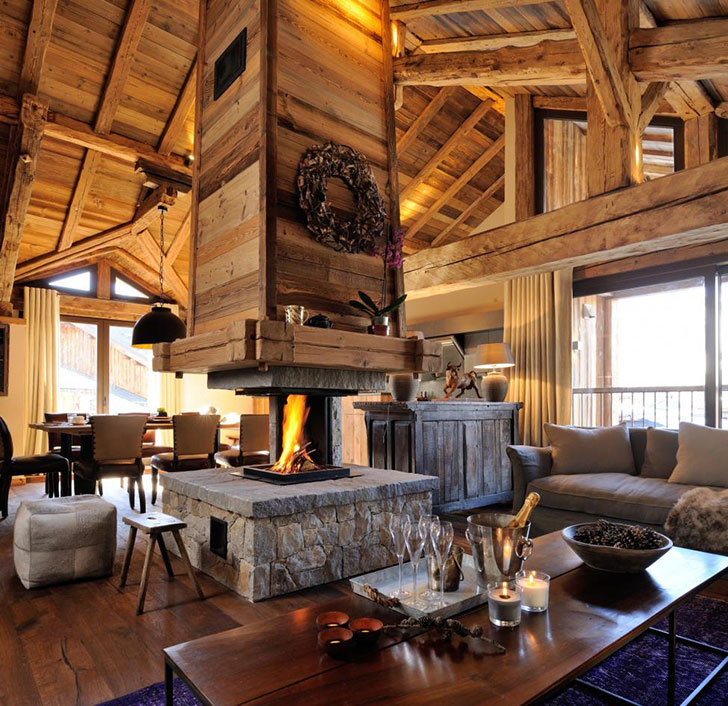The photograph captures a cozy, well-furnished living area within a house that evokes the charm of a log cabin. The room's defining feature is a central fireplace with a light gray stone base and a chimney encased in brown wood, ascending to the ceiling which peaks in a triangular shape. The ceiling and walls, all made of brown wood planks, contribute to the rustic ambiance. 

In the foreground, a coffee table made of matching brown wood is adorned with glasses, a metal bucket of champagne, candles, and a bowl of pine cones. A tan-colored couch is positioned nearby, and additional seating includes a dining table with about six chairs on one side. Off to the right of the image, a small bar can be seen with a statue of a bull, and tall sliding glass doors on either side invite natural light and provide access to the outside.

Details such as cream-colored curtains, a dark gray sofa against a window, and festive decorations like a Christmas wreath lend a homey, inviting feel to the space. The decor and setting look equally suitable for a warm living room or a serene resort hangout area, offering a welcoming retreat with its mix of wood and stone elements.